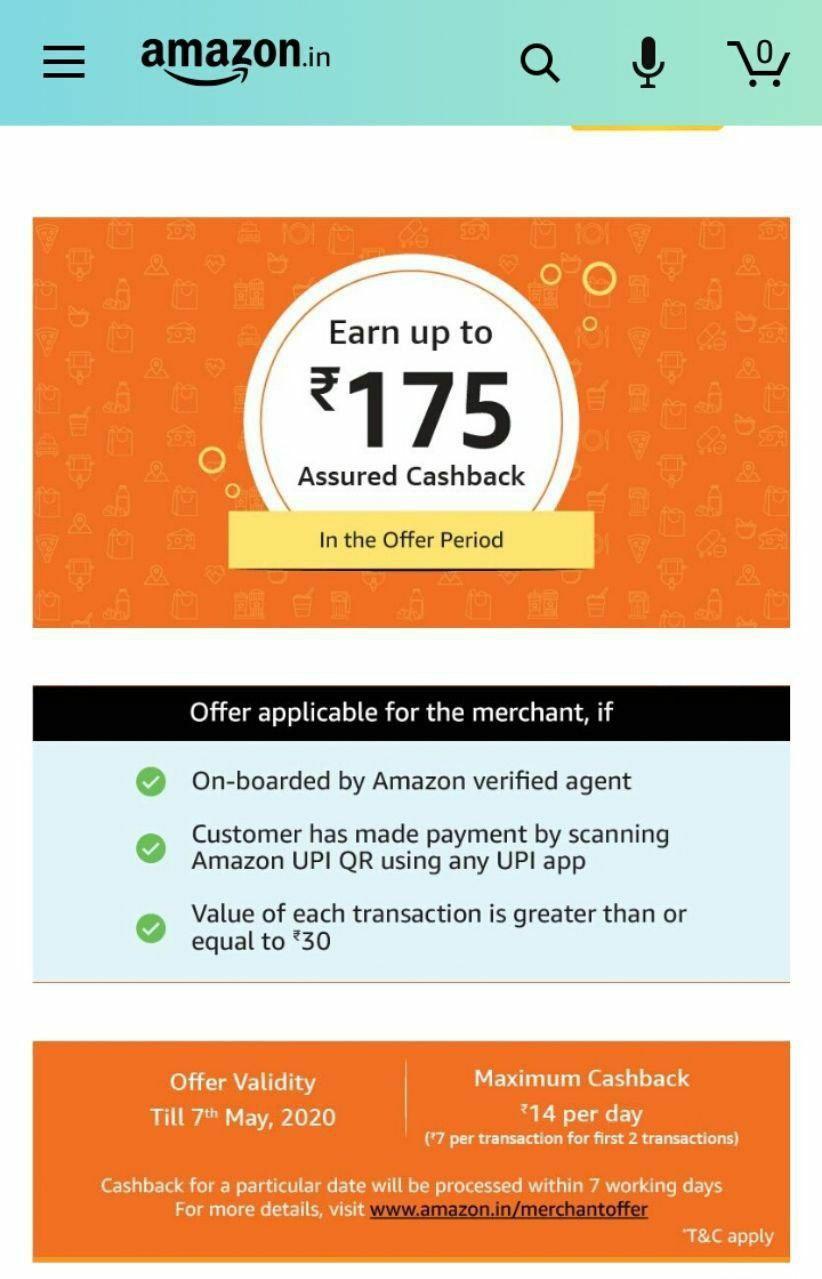Sure, here's a more polished and detailed caption for the given description:

---

The image appears to be a screenshot from the Amazon.in app, likely captured on a phone or tablet. The app interface prominently features a teal-colored border banner at the top, followed by three distinct content boxes. The top and bottom boxes have an orange background, while the middle box stands out with a light blue background and a black banner.

The primary text on the screen, prominently displayed in the largest font, reads: "Run up to ₹175 Assured Cashback," indicating a cashback offer available through the Amazon app. The black banner within the middle box states, "Offer applicable for the merchant if," followed by three criteria, each accompanied by a green checkmark, signifying that all conditions have been met.

Lastly, the bottom orange box contains crucial information about the offer's validity, stating: "Offer validity till the 7th of May 2020."

---